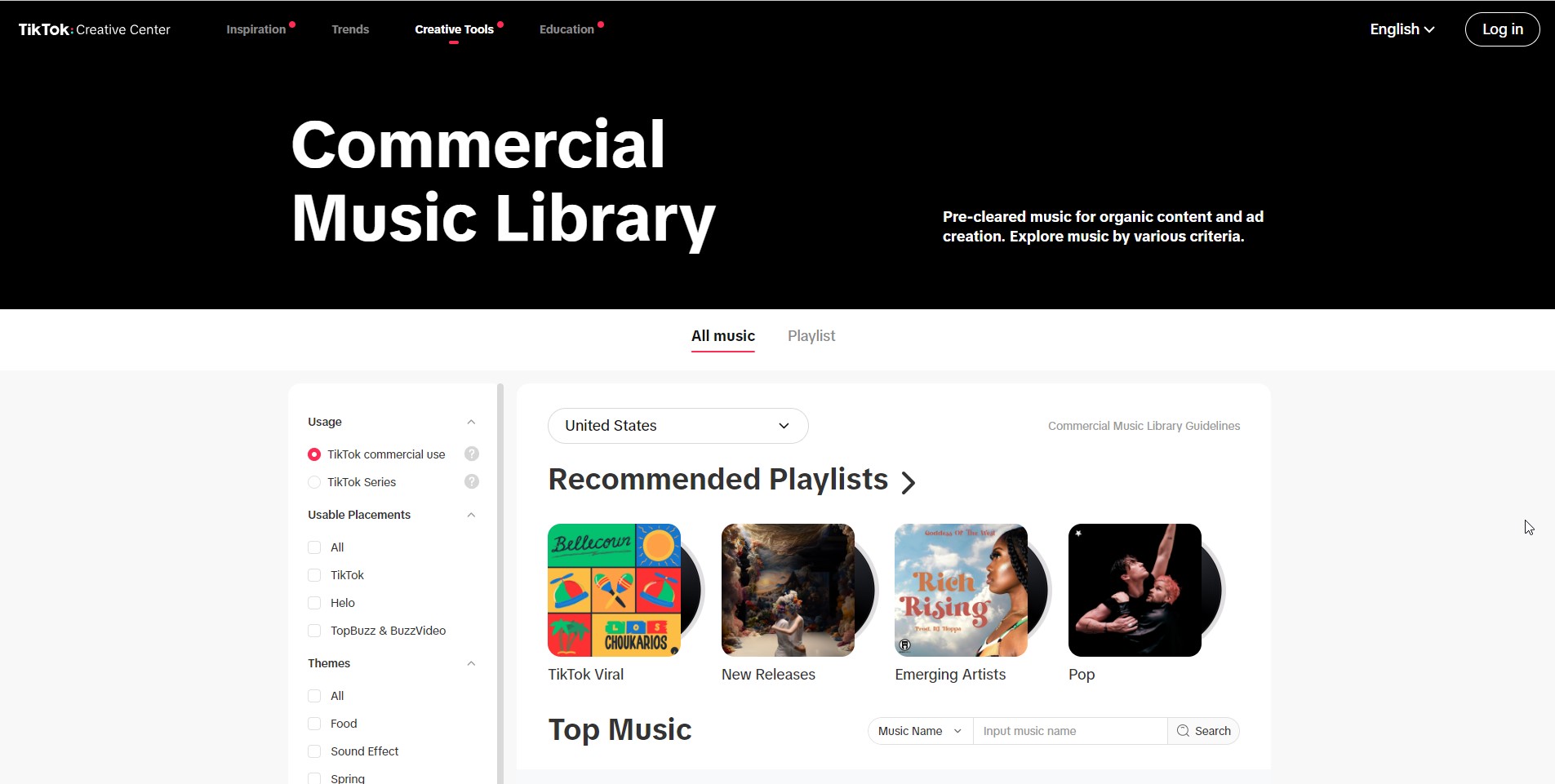This image is a detailed screenshot of the TikTok Creative Centre website. The top of the page is marked by a prominent black bar containing tiny text, which I had to zoom in to read. It displays the headings: "TikTok Creative Centre," "Inspiration," "Trends," "Creative Tools" (which appears to be underlined and selected), and "Education." To the right, there are options for language selection ("English") and a "Login" button.

Below this, in large white text, the header reads "Commercial Music Library, Precleared Music for Organic Content and Ad Creation. Explore Music by Various Criteria." The background of this section is white, predominantly featuring black text.

On the left-hand side, there is a vertical navigation bar listing categories and sections such as "Usage," "TikTok Commercial Use," "TikTok Series," "Useful Placements," "All TikTok," "Hello," "Top Buzz and Buzz Video," "Themes," "All Food," "Sound Effects," and "Spring."

To the right of this bar, there are two tabs: "All Music," which is currently selected, and "Playlist," which is greyed out. Beneath this, there are options for "United States Selected," "Commercial Music," "Library Guidelines," and "Recommended Playlists."

Four feature blocks are prominently displayed:
1. "TikTok Virals" – showcases vibrant squares and rectangles with blue, yellow, and green designs.
2. "New Releases" – features a dark, impressionist-style image that may depict a woman.
3. "Emerging Artists" – shows a rise of new talent with a close-up of a black woman with long hair.
4. "Pop" – highlights a young Caucasian man singing against a black background.

At the bottom of the image, under the "Top Music" section, there is a search function labeled "Input Music Name" and a "Search" button.